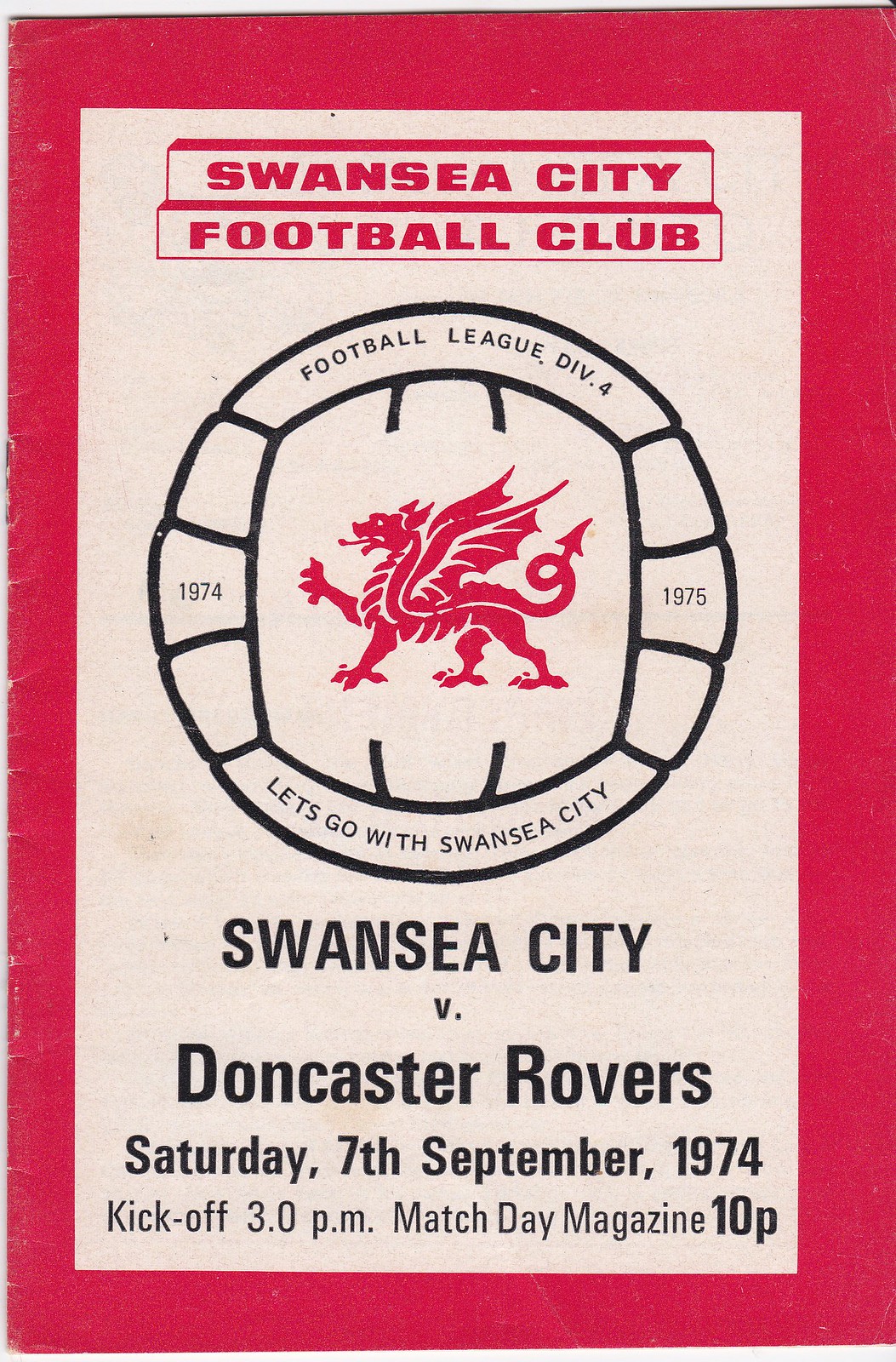This is a vintage football program poster for a match between Swansea City and Doncaster Rovers, dated Saturday, 7th September 1974, with a kickoff at 3 p.m. The program, which cost 10p, is set against a white background with a distinct red border along the top. Prominent red and pinkish-red lettering heads the poster, reading "Swansea City Football Club" in a red-outlined box. At the center, a black-outlined football features a red dragon emblem. Surrounding the football are texts denoting "Football League Division 4" at the top and the years "1974" on the left and "1975" on the right in light gray letters. At the bottom of the football is the rallying cry, "Let's go with Swansea City." Below the football image is the match information: "Swansea City v. Doncaster Rovers, Saturday, 7th September 1974, Kickoff 3 p.m., Match Day Magazine 10p."